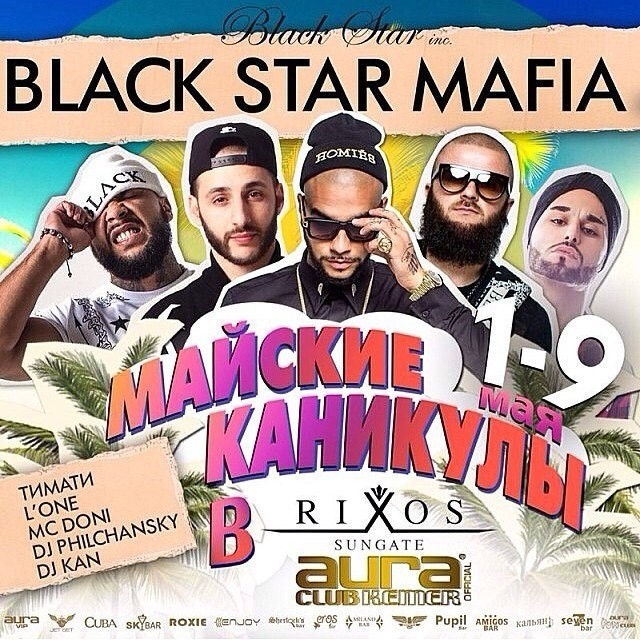The image is a promotional flyer for a music event, featuring five men from the chest up. The top of the flyer displays the text "Black Star Inc." and "Black Star Mafia," layered over a ripped cardboard-effect background. Behind the group is a backdrop of yellow plants. The five males are all facing forward, with varied attire: the man on the far left wears a white beanie with black letters and a white shirt, has a full beard, and is grimacing. The second man from the left wears a black ball cap and a black shirt, also sporting a full beard. Centered is a bald man with facial hair, wearing black sunglasses, gold jewelry, a black long-sleeve button-down shirt, and a black beanie. Next to him, the center-right man has short cropped hair, glasses, a beard, and a black shirt. The person on the far right is wearing a turban. Below the men, there is text in what appears to be Russian, along with the date range "1-9 March." The advertisement is sponsored by Rio Sungate, Aura Club, and Kimmer Official, with a list of performers, including names like DJ Kan and MC Dhoni, displayed on the left side. The flyer features a color palette of tan, orange, light purple, purple, off-colored red, and various black and white lettering. The entire composition suggests a digitally created flyer aimed at promoting a music event.